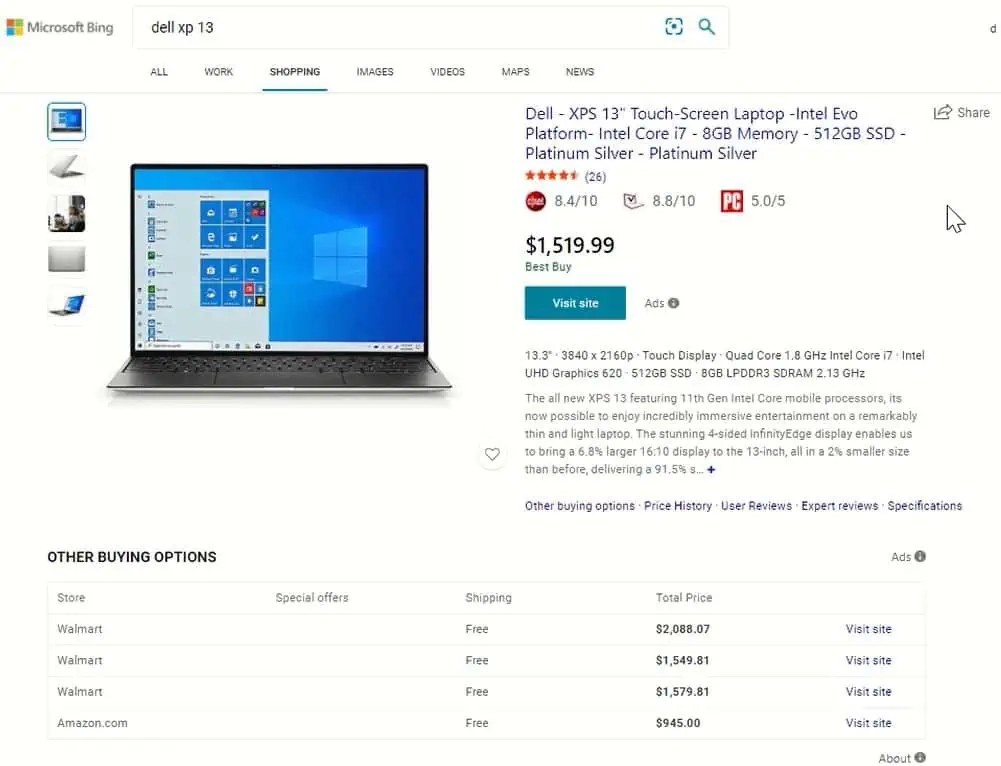A detailed screenshot of a Microsoft Bing shopping website displaying a Dell XPS 13-inch touchscreen laptop. At the top left, the website header prominently reads "Microsoft Bing," followed by a search bar pre-filled with "Dell XP13." Below the search bar are category tabs: All, Work, Shopping (highlighted), Images, Videos, Maps, and News.

In the main section, there's a close-up image of the Dell XPS 13 laptop, with five additional thumbnail views on the left side. To the right of the laptop image is a detailed description and pricing information. The title of the product reads, "Dell XPS 13-inch Touchscreen Laptop, Intel Evo platform, Intel Core i7, 8GB Memory, 512GB SSD, Platinum Silver/Platinum Silver."

The listing also displays customer ratings and scores: 
- 4.5 stars (26 reviews)
- An 8.4/10 rating inside a red circle
- An 8.8/10 rating next to another symbol
- A red square labeled "PC" with a score of 5.05/5

The laptop is priced at $1,519.99. Below the price, in blue text, is a link to "Best Buy," accompanied by a blue "Visit Site" button. The word "Ads" appears in gray to the right. At the bottom of the page, there's a footer menu with further navigation options.